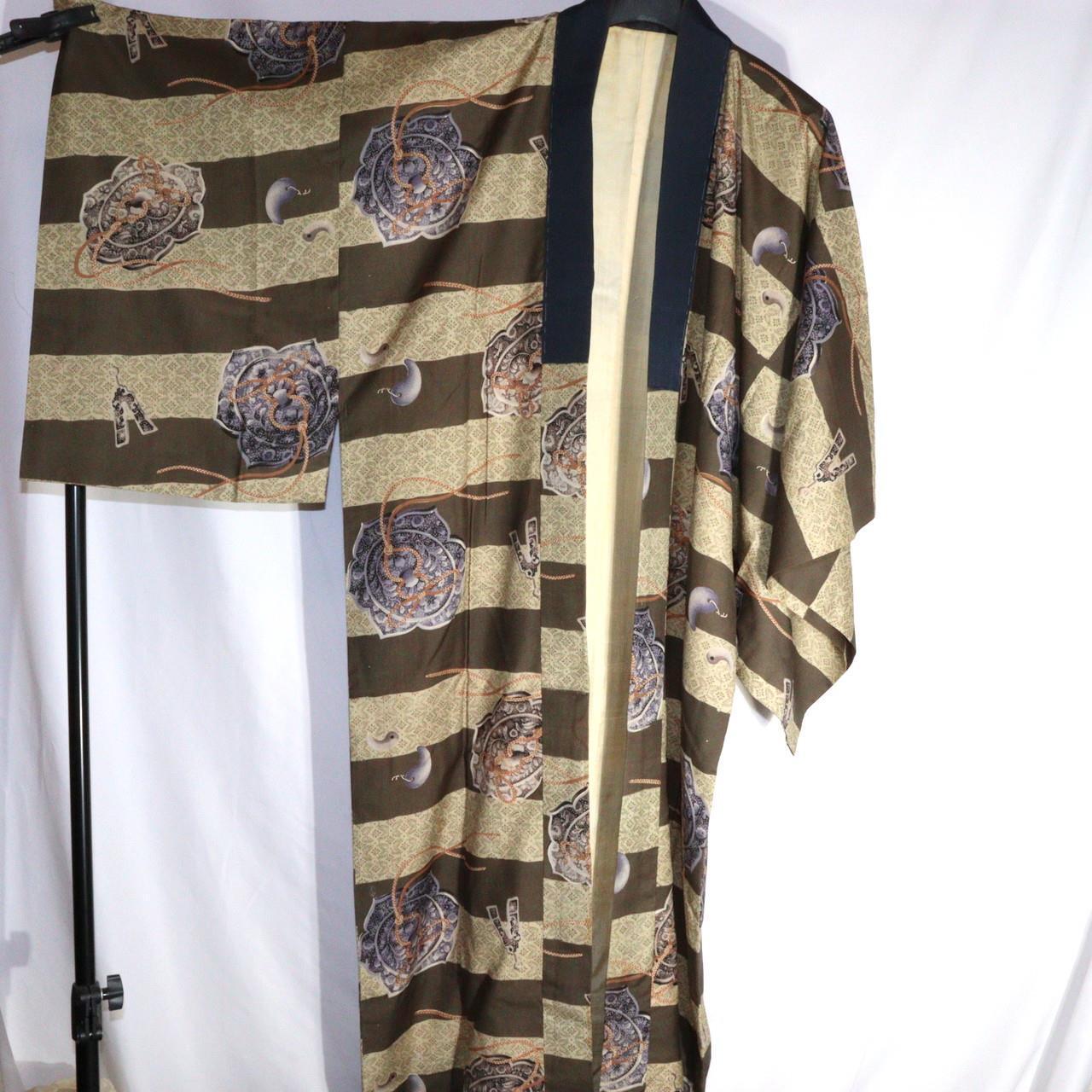This image features a kimono-like robe with a lightweight, thin texture, primarily light brown and beige in color. The robe is adorned with designs resembling flowers, some in blue and others in beige, adding a decorative touch. The upper part of the robe, including the collar, is blue, while the bottom half maintains the beige hue. The sleeves of the robe are notably long, akin to those of a kimono.

The robe is displayed in front of a white curtain, which creates a soft, neutral background. A black stand, visible on the left side of the image, holds up the robe. The stand includes a black pole with a tightening mechanism, securely clipping the left sleeve of the robe. The right sleeve of the kimono is raised, while the left sleeve hangs in a more relaxed position.

Horizontally along the garment, there are alternating solid brown and tan stripes, forming a consistent pattern across the torso and down towards the feet. Interspersed among these stripes are intricate figures of gray medallions and yin-yang symbols, rendered in gray, silver, and white. These elements contribute to the robe's distinct and sophisticated design.